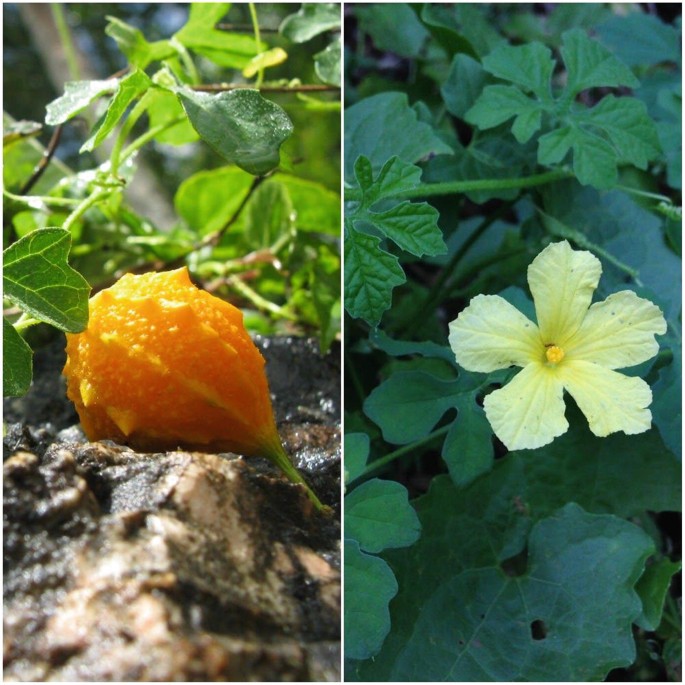The image is a square composition featuring two color photographs in portrait orientation, separated by a narrow white line down the center. Both photographs are of the same size and shape. The left photograph showcases an orange fruit, likely a jackfruit, positioned centrally with a rough, pointed outer skin. The fruit is nestled among dark green leaves at the top and is set against a backdrop of brown and gray rocks. The jackfruit has a pointed end facing the bottom right, transitioning into a rounded, bulbous top on the left side.

The right photograph captures a pale yellow hibiscus bloom near the right center of the frame. The viewer is offered a perspective looking down into the heart of the blossom, revealing a central round yellow area. The hibiscus has five petals radiating outward in a star-like formation. The flower is set against a background of dark green, tightly packed foliage, enhancing the details of the bloom. The overall style of the imagery is photographic representational realism.